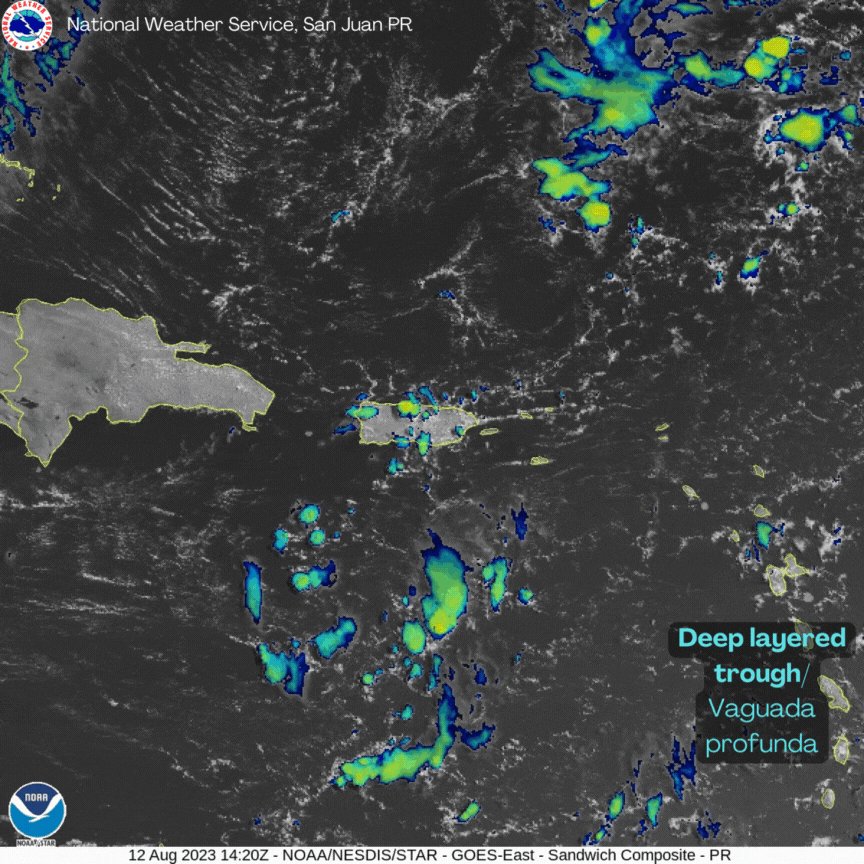The image is a detailed National Weather Service projection for San Juan, Puerto Rico, dated August 12, 2023, displaying a weather forecast. The projection features a gray outline of Puerto Rico and adjacent islands, highlighting the presence of bodies of water. Various colored regions, primarily in bright blue, green, and yellow, depict temperature zones and weather fronts. Prominently, a weather front moving through the area is represented by these colors. Notable text on the image includes "National Weather Service, San Juan, Puerto Rico" at the top left, "Deep Layer Trough, Vagunda Profunda" on the right, and additional annotations at the bottom left, including "Nora" and the timestamp "1420Z". Furthermore, acronyms and data descriptors such as "NOAA/NESDIS/star - GOES-east-sandwich composite-PR" underscore the technical nature of this satellite weather forecast, which predicts an incoming weather system, possibly a hurricane, advancing toward Puerto Rico.